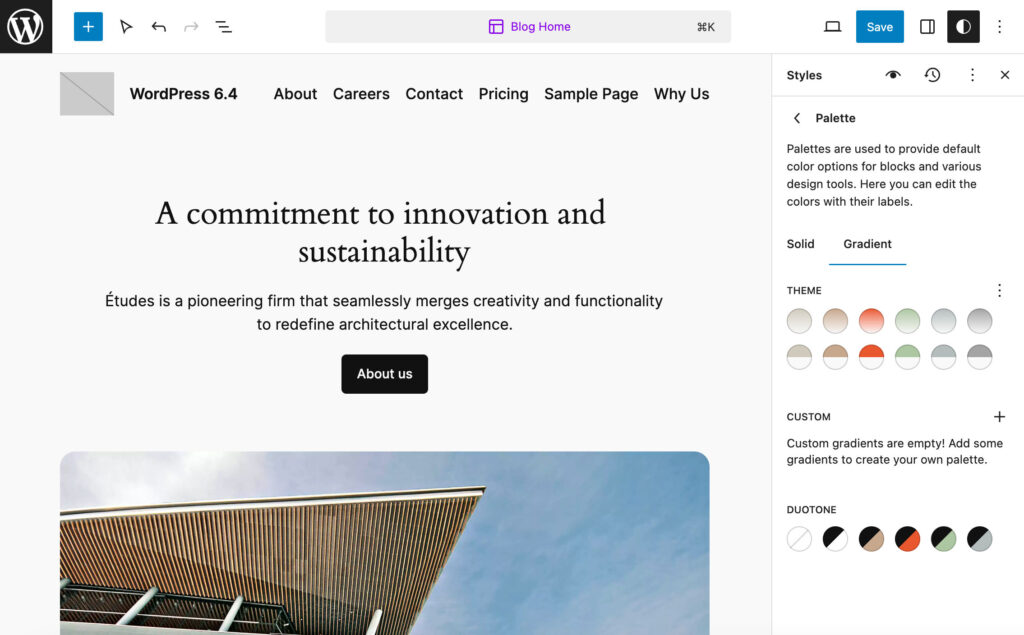The image depicts the interface of a WordPress website. At the top right corner, there is a distinctive WordPress icon consisting of a black square with a white circle and a white "W" in the center. Adjacent to it, there are several icons including a plus icon, an arrow icon, and a back icon. The navigation bar includes links labeled "Blog Home" and "PC", with options to save and switch between dark mode and bright mode.

The displayed interface is of WordPress version 6.4. The top menu includes links titled "About", "Careers", "Contact", "Pricing", "Sample Pages", "Why Us", and "A Commitment to Innovation and Sustainability". Below this, there is a statement written in another language, followed by a descriptive sentence in English: "Etuse is a pioneer firm that seamlessly merges creativity and functionality to redefine architectural excellence".

Further down, there is a section titled "About Us" and at the bottom of the image, a photograph of an architectural structure is visible. On the right side, there are options for "Styles" and "Palettes", with sub-options for "Solid" and "Gradients" representing different color choices, as well as a "Custom" option. There seems to be a button labeled "Button", possibly for additional customization features.